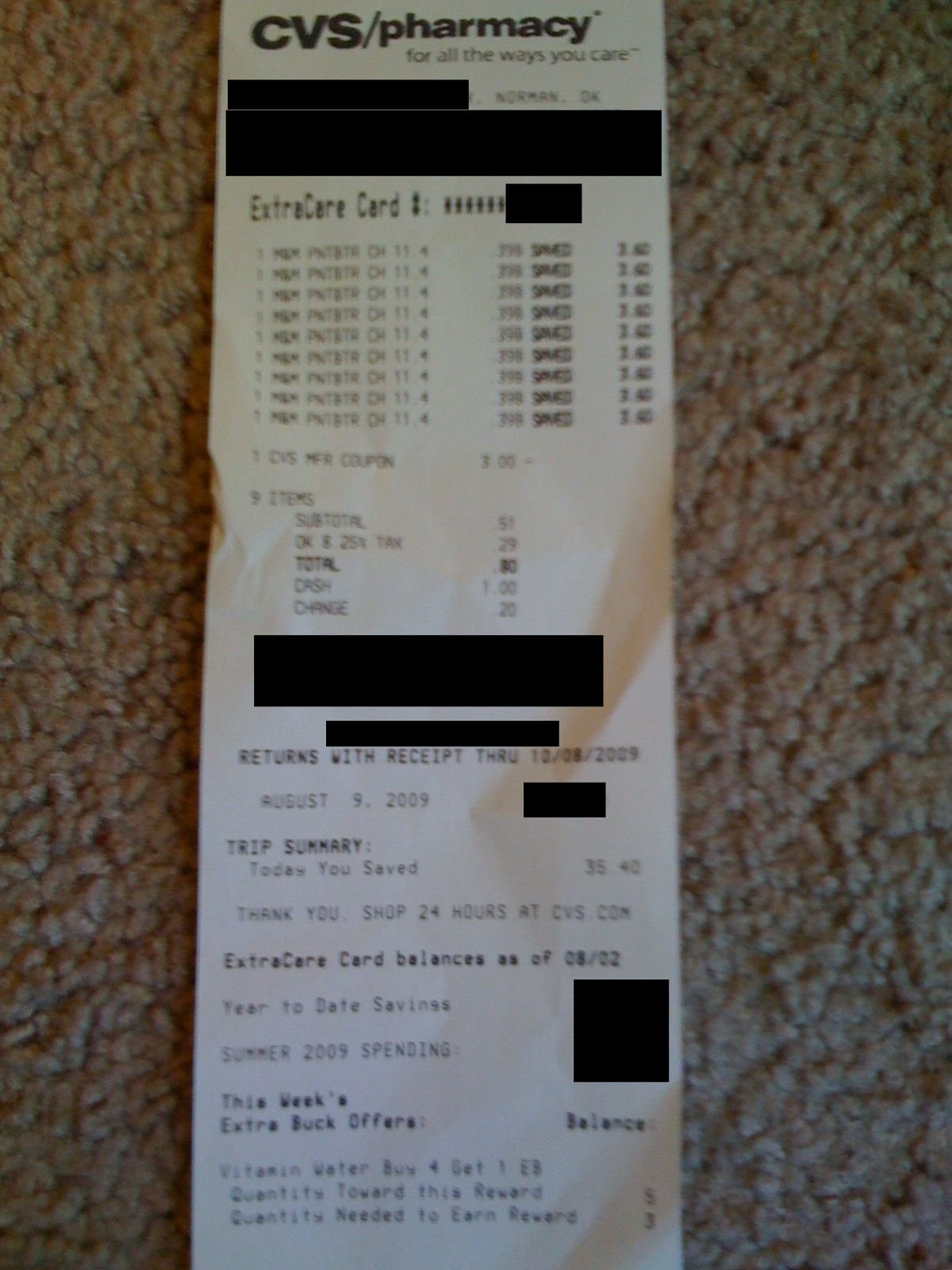A color image of a CVS pharmacy receipt taken against a tan, bumpy carpet background, possibly with grayish or white tones. The top of the receipt prominently displays "CVS / Pharmacy" in bold, followed by the tagline "For all the ways you care" in non-bold print. Certain sections of the receipt are obscured by black rectangles, likely to conceal personal information. The visible text includes "extra care card" and an array of asterisks, indicating censored information. The transaction details show a subtotal of approximately 50 cents, with an additional tax of 29 cents, culminating in a cash payment of one dollar and 20 cents in change given. The receipt notes a returns policy valid through October 8, 2009, and contains a summary indicating savings of $35.40 and additional information about year-to-date services and ExtraCare balance. However, some of these sections are too blurred to read clearly.